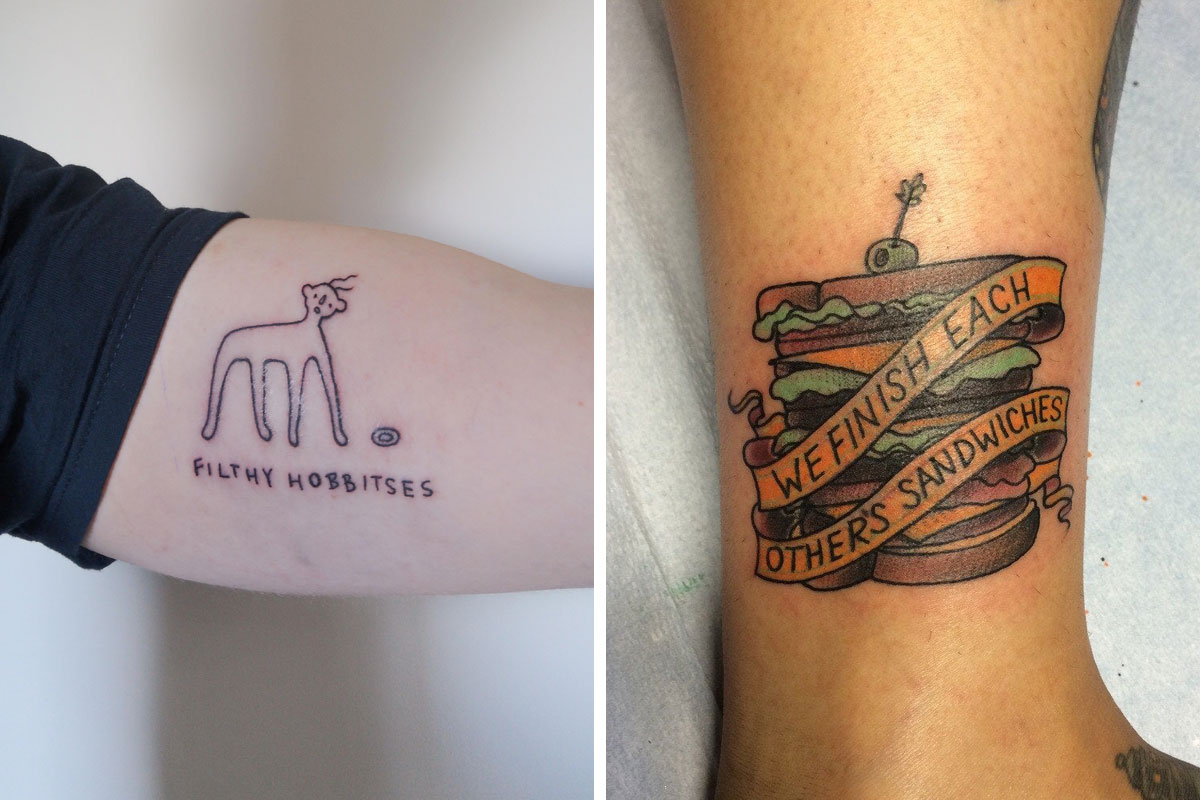The image displays two panels, each showcasing a unique tattoo on different body parts. The left panel features the inner arm of a person with very fair skin, wearing a black t-shirt with the sleeve rolled up. The tattoo is a simplistic, cartoon-like drawing of a four-legged figure outlined in purple, with two little hairs on its head. Beneath the figure, in purple writing, is the phrase "Filthy Hobbitses," along with a small, circular object resembling a ball. The background behind this arm is white. The right panel depicts the inner left leg, likely near the ankle, of a person with slightly tanned skin. The tattoo here is a vibrant, multi-layered sandwich complete with green lettuce, colored meat, and distinguishable bread slices. Atop the sandwich sits a green olive skewered by a fancy toothpick. The scene is framed by a banner that reads "We finish each other's sandwiches," all set against a white background.